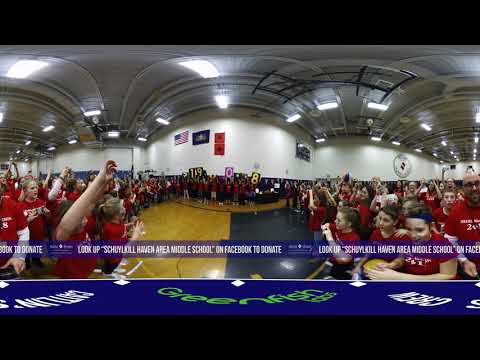This 360-degree photo captures a lively scene of students at Schuylkill Haven Area Middle School, gathered in a gymnasium that doubles as an auditorium. The students, all adorned in matching red shirts with indistinguishable white text, fill the space with an exuberant energy. Some of them hold up signs displaying the numbers "1908". The gymnasium floor is divided, with the left side showcasing a tan or brown wood finish and the right side covered in a navy blue surface. In the backdrop, a white wall supports an American flag among other hanging items. Above, white metal support beams and scattered lights frame the ceiling, adding to the structured chaos of the scene. At the very front and bottom of the image, bold green letters spell out "Green Fish" on a cobalt blue background, accompanied by a scrolling message urging viewers to look up Schuylkill Haven Area Middle School on Facebook to donate. The photo also features one visible adult positioned on the far right, amidst the sea of cheering and smiling students.